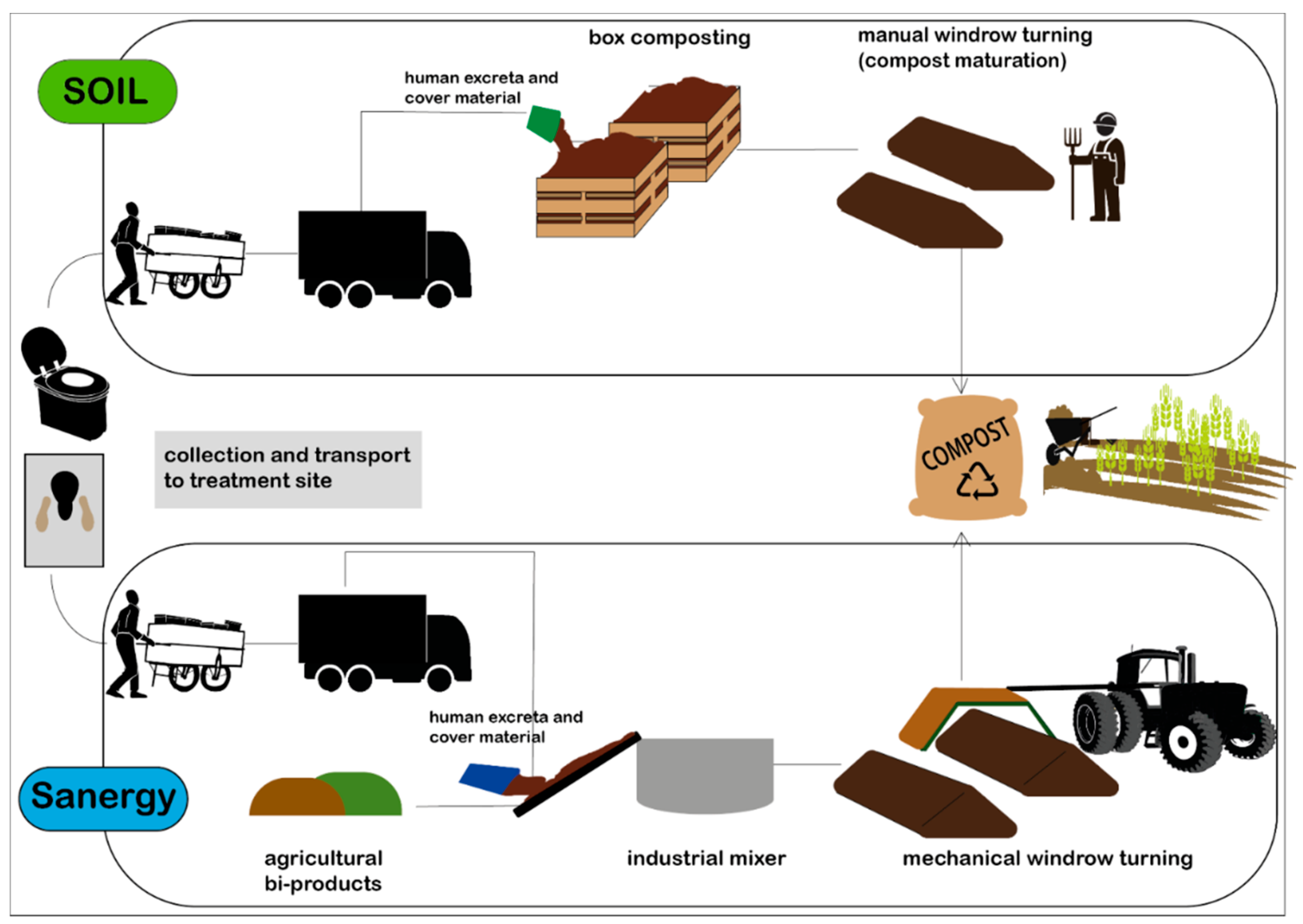This detailed diagram, rendered in black on a white background, illustrates two methods for processing human waste into usable compost for agricultural purposes. The top part of the illustration, labeled with a green text bubble, follows a path where human excreta, combined with cover material, is transported via truck to a box composting system. Here, the waste undergoes manual windrow turning and compost maturation, ultimately being bagged as compost. The bottom section, marked as "Sanergy," denotes an alternative method using human excreta and cover material mixed with agricultural byproducts in an industrial mixer. This mixture then goes through mechanical windrow turning before also being processed into compost. The diagram features various stages of the composting process, including images of a toilet, a person transporting waste, trucks, composting vats or boxes, and final applications in fields using a tractor to spread the compost. Overall, the diagram serves as an informative guide on transforming human waste into valuable fertilizer through different composting techniques.